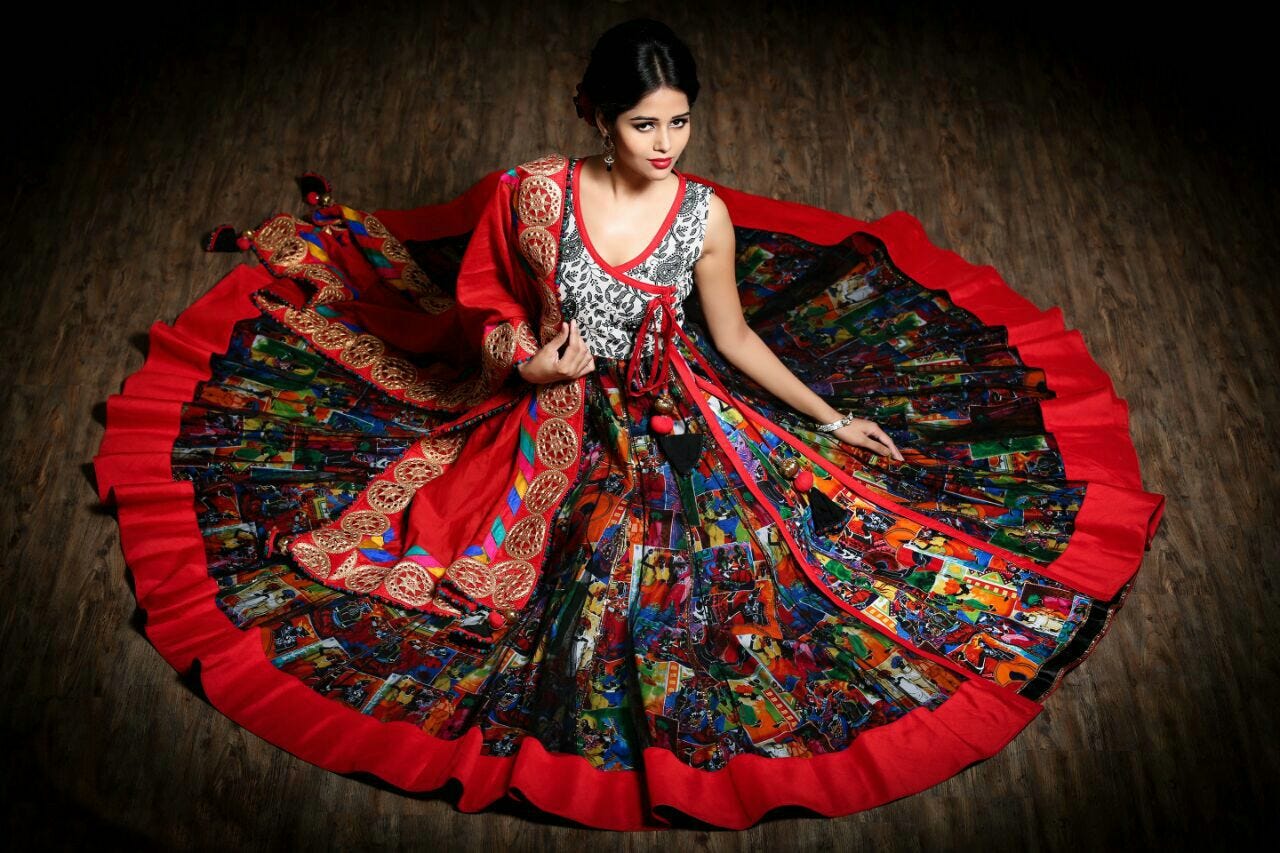In this vibrant and intricately detailed photograph, a young woman with pale skin and black hair, styled back, wears an elaborate and culturally rich dress that radiates a sense of tradition and celebration. Her striking look is completed with bright red lipstick and a silver bracelet on her wrist. The upper half of her outfit is a sleeveless, wrap-around top, predominantly white adorned with gray botanical and paisley motifs, accented by a red trim around the chest and a red tie closure. Draped over her right shoulder is a richly adorned red cloak with heavy ornamentation featuring gold round medallions, star designs, and multicolored blocks of blue, yellow, pink, and turquoise. 

Seated gracefully on a wooden surface—dark near the edges but brown towards the center—she spreads out her voluminous skirt in a perfect, circular display around her. The skirt, solidly red with an intricate sequence of images and motifs in dominant hues of black and blue, showcases a patchwork of colorful pieces framed by a red hem. The dress's vivid and detailed design, paired with the wooden backdrop, creates an almost surreal and vividly colorful tableau that might seem almost computer-generated at first glance.